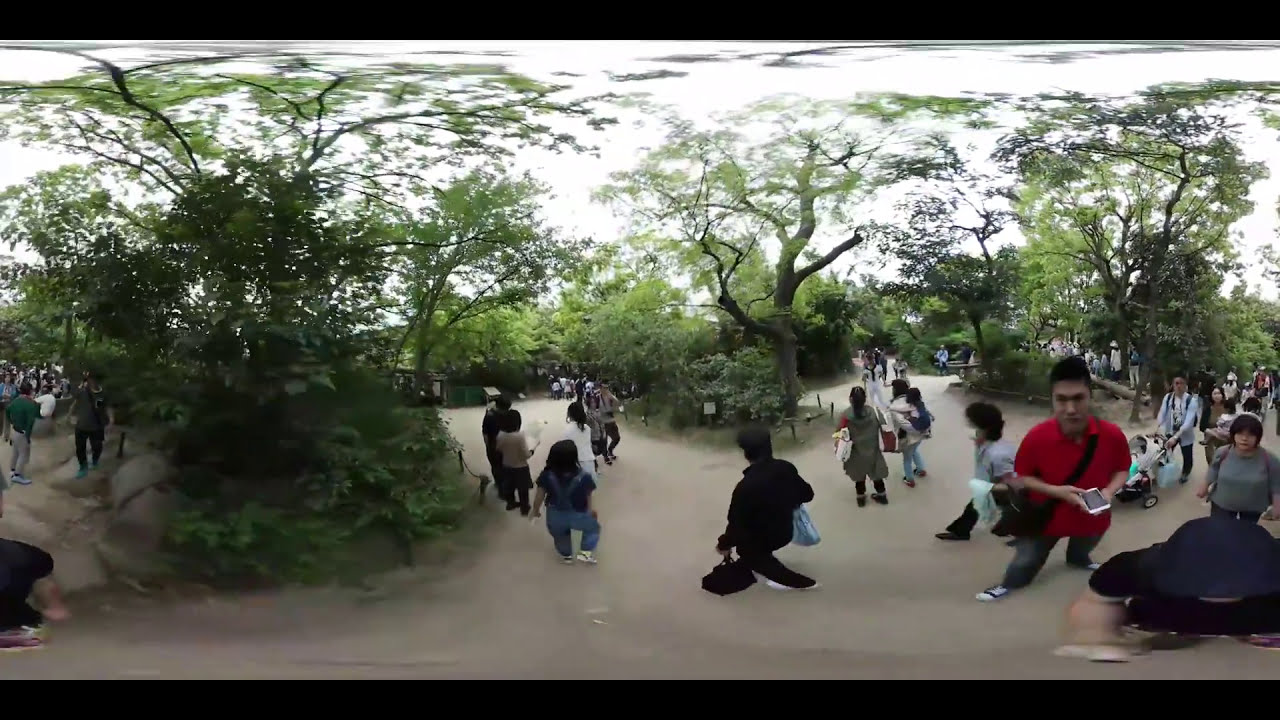This image captures an outdoor scene in what appears to be a crowded, family-friendly area, possibly a zoo or a public park. The picture is slightly distorted as if spliced together, giving a panoramic view of the setting. Central to the image is a stone walkway bustling with various people, including a young man in jeans and a red Polish shirt carrying a backpack. Another noticeable figure is someone pushing a child in a stroller. The crowd is diverse, with individuals carrying children, purses, other bags, and more backpacks.

The surroundings showcase abundant greenery with several clumps of trees and shrubs featuring brown trunks and lush green foliage. The ground appears tan-colored, though the haziness of the photograph makes it hard to discern other specifics. The overall brightness suggests a midday setting, though details about the weather remain ambiguous due to the light saturation. The photo, measuring approximately 8 inches wide by 5 inches tall, is framed by black borders at the top and bottom, further accentuating its panoramic nature. Multiple colors are visible throughout the scene, including black, gray, green, red, light blue, yellow, and tan, contributing to the dynamism of this lively outdoor environment.